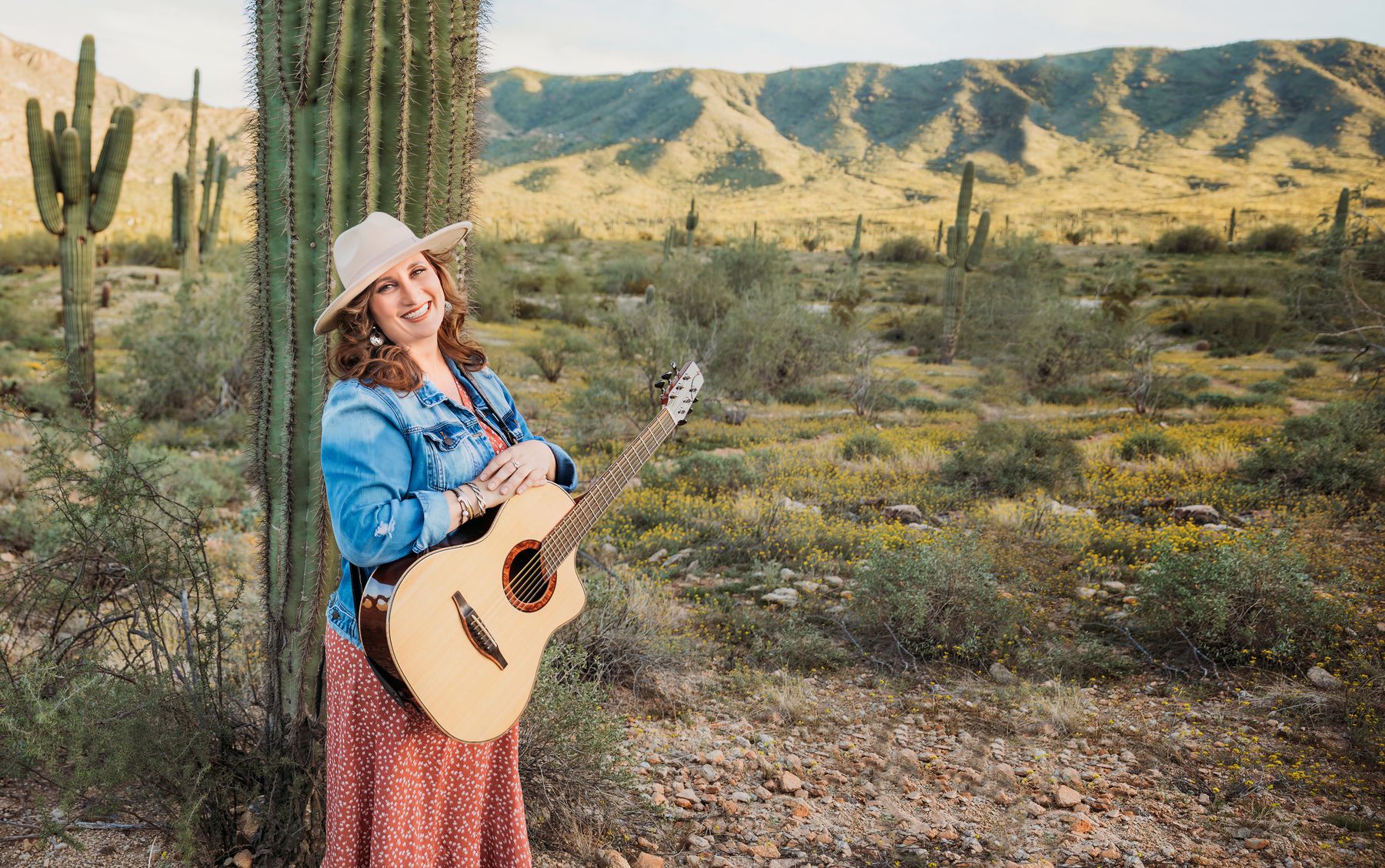A detailed photograph captures a cheerful woman with a light white complexion, standing prominently in a vast, rocky desert landscape. She is wearing a tan Panama-style hat that shades her reddish brown, shoulder-length curly hair. Her attire includes a light blue denim jacket draped casually over a salmon-colored shirt paired with a salmon-colored skirt adorned with little white dots. She accessorizes with two visible bracelets on her right wrist. The woman exudes a warm, inviting smile as her folded arms rest atop the body of her light tan acoustic guitar, which hangs around her neck.

Behind her, a large cactus stands tall, with several other cacti and desert plants scattered about, some resembling green tumbleweeds. The desert floor is a textured mix of sand, gravel, rocks of various colors including brown and dark gray, and native brush. In the distance, a range of tan and green mountains extends across the horizon, transitioning into a pale, grayish sky. The shadowing in the image appears slightly mismatched, suggesting the possibility that the woman might have been pasted into the scene. The overall atmosphere conveys a serene, yet vibrant desert oasis, potentially reminiscent of regions like Arizona.